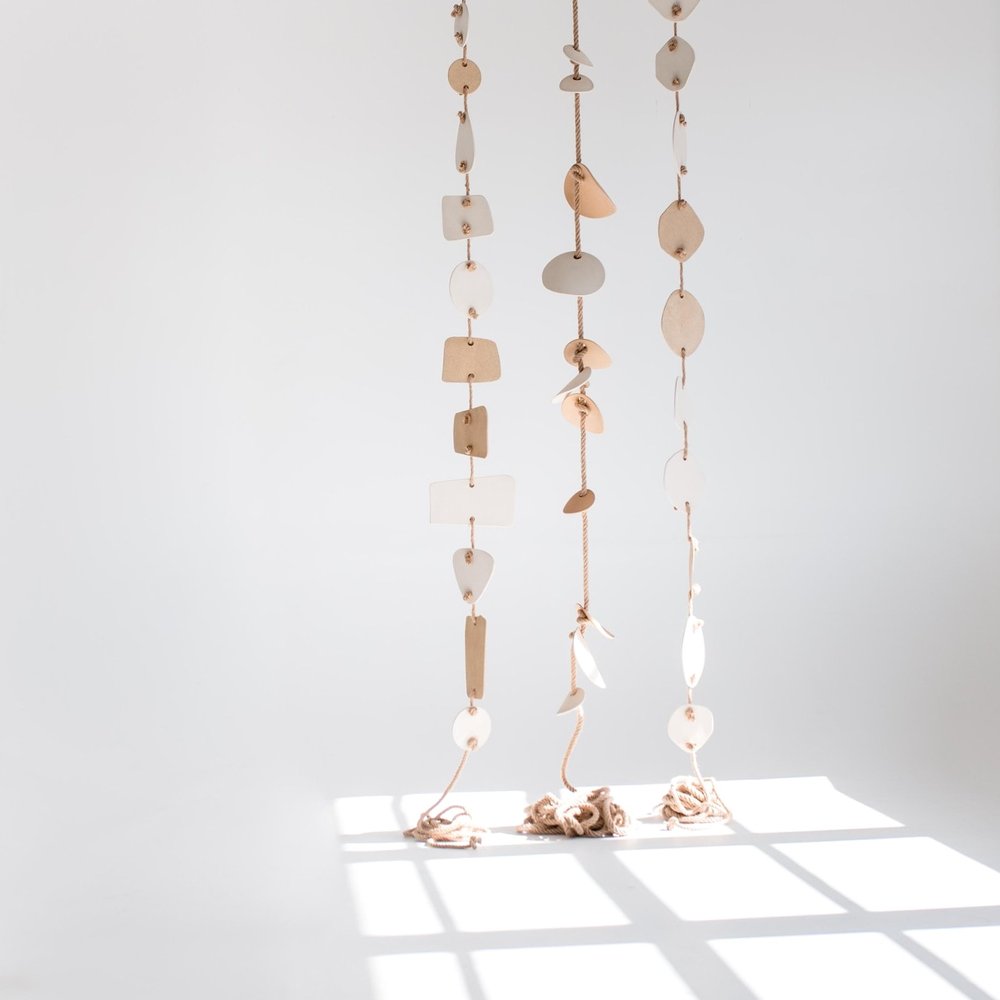The image captures an artful installation set against a light gray backdrop, which could be a studio setting. Soft sunlight streams through an unseen window, casting a grid-like pattern of white squares—formed by the window panes—symmetrically across the floor from the bottom right to the top left of the frame. At the top of this shadowy reflection, a bundle of thick rope or jute descends, disappearing out of the frame at the top. This rope branches into three strings threaded with a series of objects including shells, possible metal pieces, wood, tile, and perhaps shell fragments, all showcasing a palette of neutral colors—whites, grays, tans, and browns. These objects are meticulously knotted at intervals on the strings, which lend the overall arrangement a minimalist yet modern aesthetic. The strings cascade gracefully, suspending the varied pieces in an elegant, almost wind chime-like fashion. The interplay of shadow and light, combined with the textured materials, creates a visually captivating and serene composition.